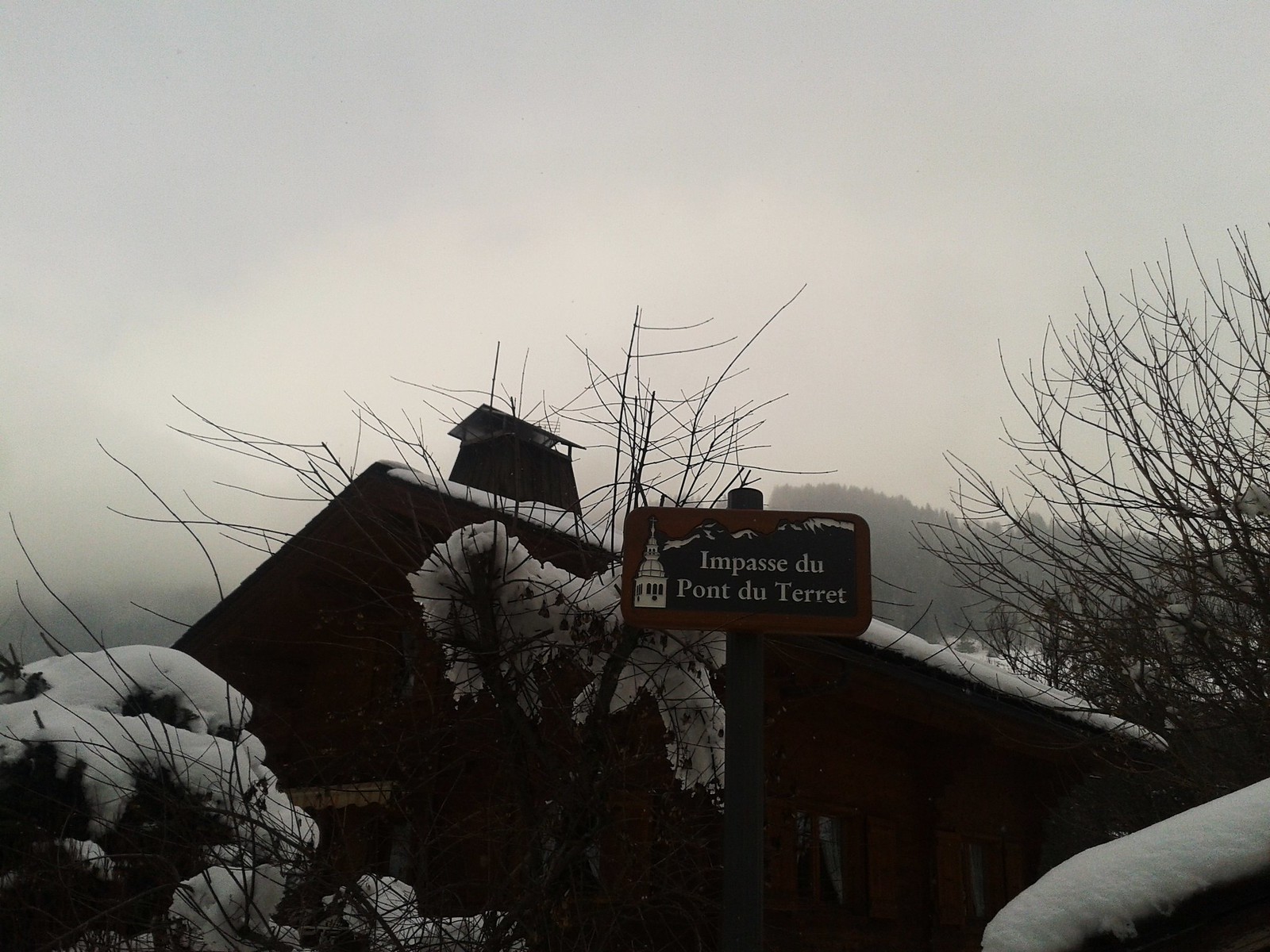A photograph captures a wintry outdoor scene dominated by an overcast, gray sky, lending a dark and foggy atmosphere to the image. In the distant horizon, a dense forest of barren trees, stripped of leaves and capped with snow, stretches out. In the foreground stands part of a house, likely a log cabin, with a chimney on its snow-covered roof. Surrounding the house, leafless bushes and trees are also blanketed in snow. Prominently positioned in front of the house is a wooden post bearing a small brown sign that reads "Impasse du Pont du Terret." This sign includes a white drawing of a small structure. The stark, snowy landscape is tinged with a hint of blue from the distant mountains or hills, creating a serene yet desolate winter scene.